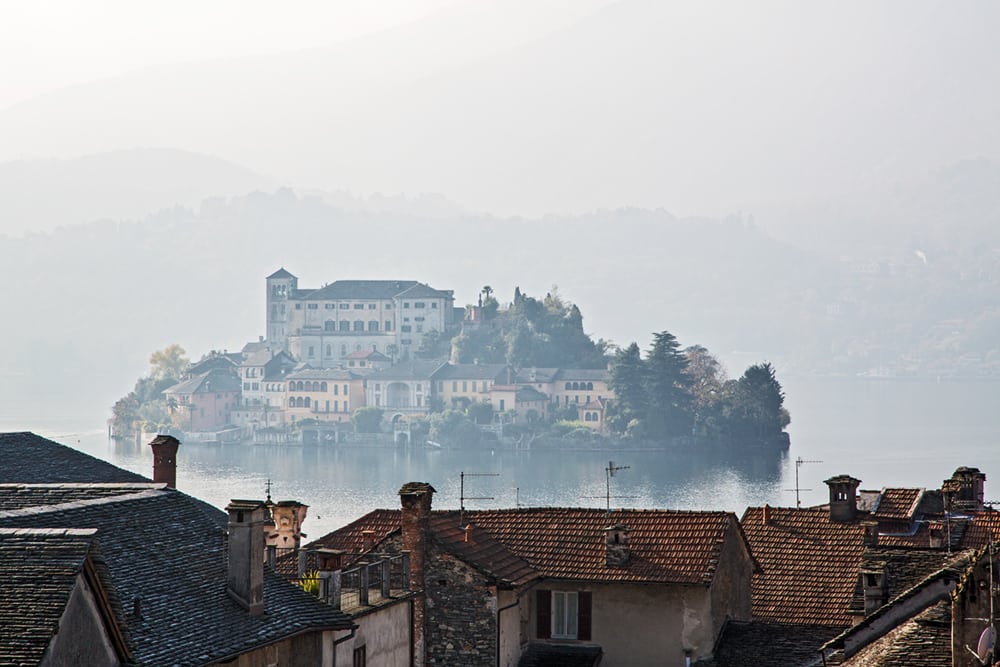In this photograph, we see a picturesque scene featuring an island situated in the middle of a large body of water. The island is adorned with multiple buildings, including a dominant, mansion-like main structure surrounded by smaller, yet significant, residence-sized edifices, all nestled amidst lush trees. The island, enveloped by water, suggests accessibility likely only by boat, adding to its secluded charm. In the foreground, the image captures the tops of five older, perhaps European-style houses with tiled roofs, chimneys, and antennas, hinting that this scene may not be in America. Dense fog blankets the background, partially obscuring layers of hills or mountains, contributing to an ethereal and serene atmosphere. The contrast between the opulent and vividly maintained island structures and the more worn and modest houses in the foreground adds a layer of narrative to this scenic vista.